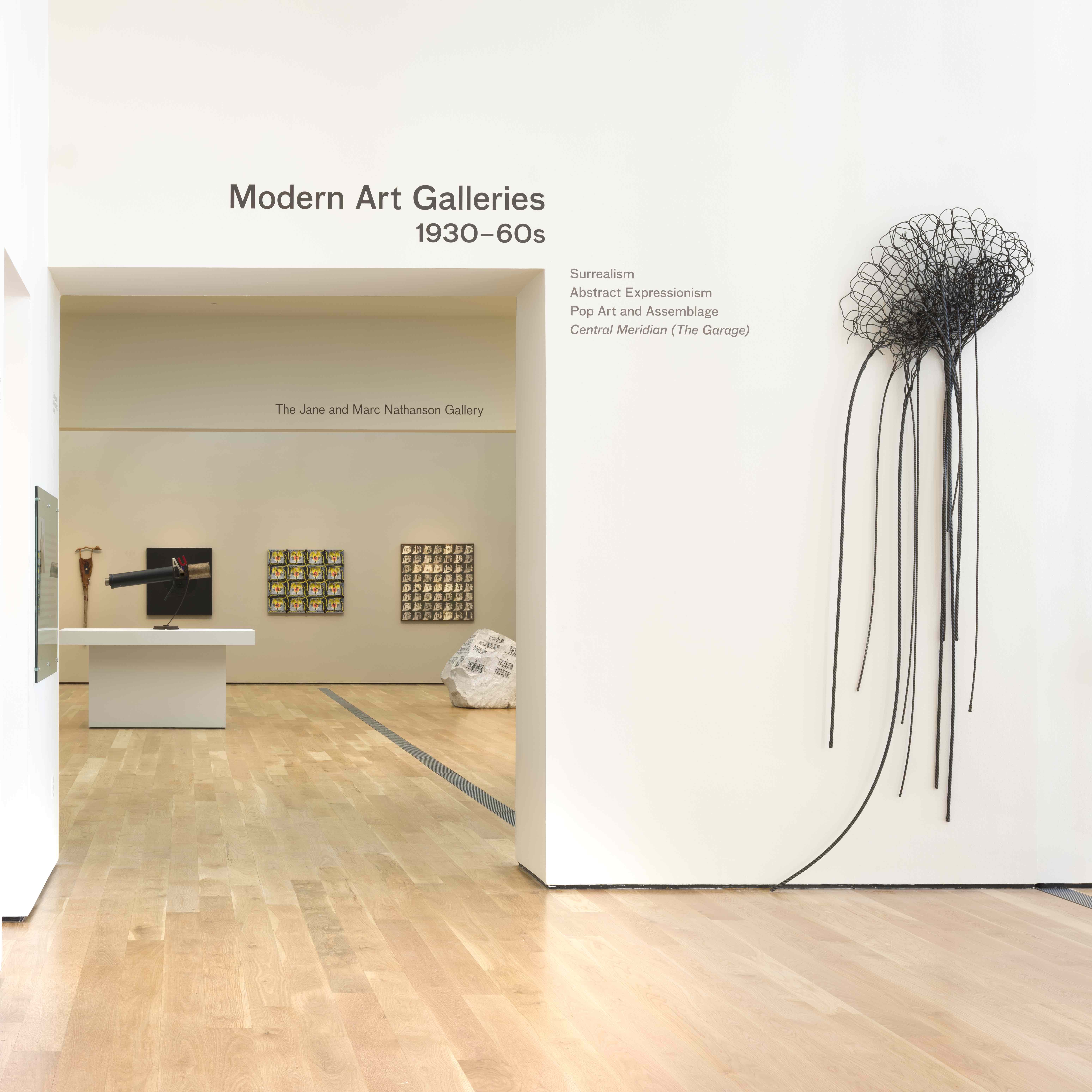The full-color vertical photograph captures an indoor scene set in an art gallery lit by artificial light. The gallery features light brown, polished hardwood flooring with two distinct grey lines running across it, potentially marking exhibit boundaries. A white wall dominates the foreground, offset by an open archway to the left. Above this archway, black text reads, "Modern Art Galleries, 1930 to 60s," and to the right of the doorway, additional black text lists, "Surrealism, Abstract Expressionism, Pop Art and Assemblage, Central Meridian (The Garage)."

To the far right on the white wall, there's an abstract sculpture resembling a jellyfish, crafted from black wire or rope with long, flowing strings that dangle towards the floor. Beyond the archway, another room is visible, hosting more artworks on its walls and featuring a white countertop with objects on it. Notable in this distant room is a large white boulder and a telescope on a white pedestal, beneath a sign that reads, “The Jane and Mark Nathanson Gallery.”